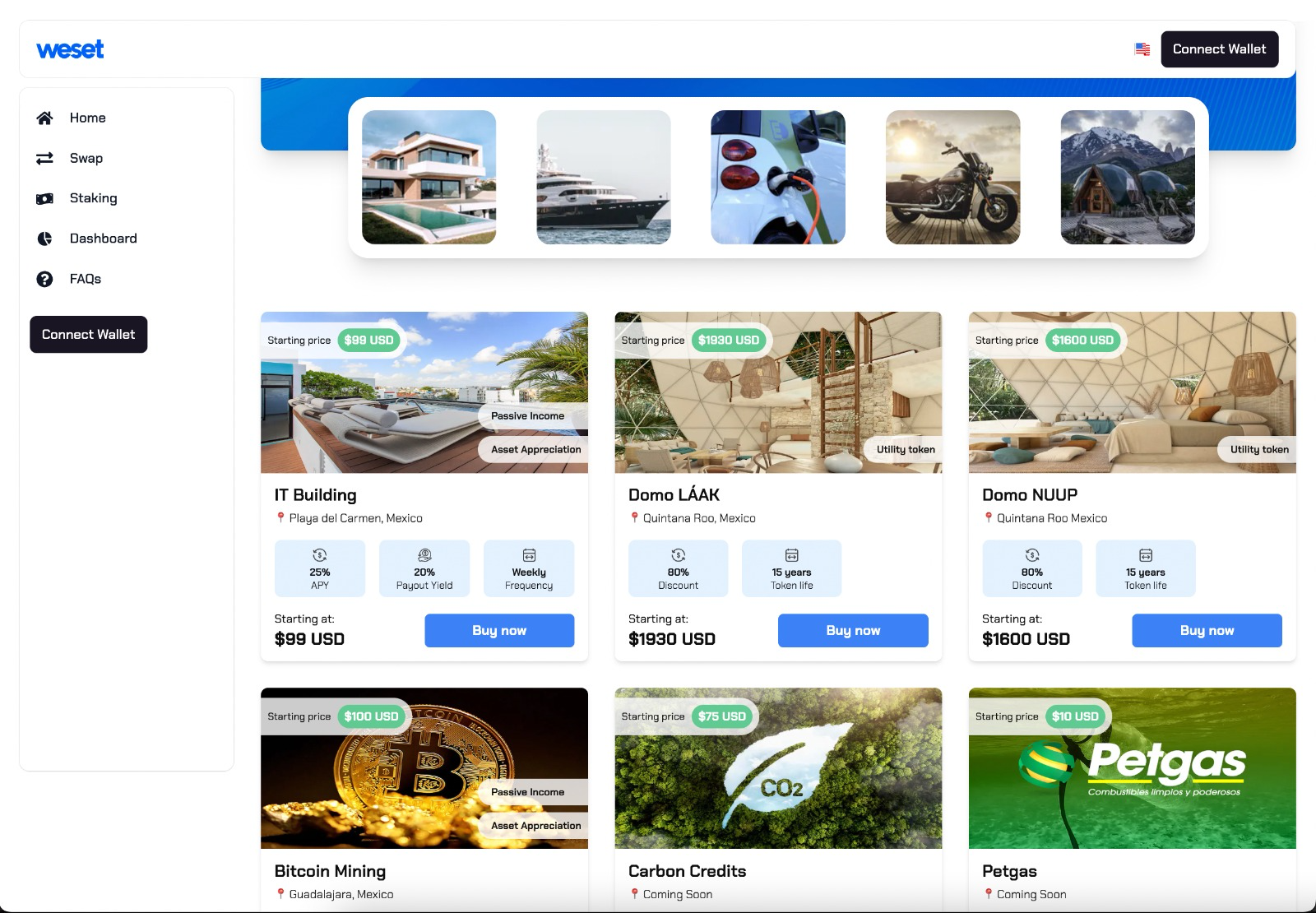This screenshot depicts a webpage from a website named WESET, shown on a desktop or laptop computer. The website appears to cater to cryptocurrency users, as evidenced by the prominent "Connect Wallet" button in the upper right corner, next to an American flag icon suggesting language or regional settings. The left-hand column features a navigation menu with several options: Home, Swap, Staking, Dashboard, FAQs, and an additional "Connect Wallet" button.

The main content section of the site showcases various items and services available for purchase or bidding using cryptocurrency. Among these offerings are "IT Building," available starting at $99 USD, "Domo Lock," starting at $1930 USD, and "Domo Noop," starting at $1800 USD. Additional sections feature opportunities in Bitcoin Mining, Carbon Credits, and Pet Gas.

Based on this layout and the items listed, the website appears to function as a marketplace where users can either bid on or directly purchase a variety of goods and services using cryptocurrency. The detailed nature of the options suggests a platform designed for users familiar with digital currency transactions.